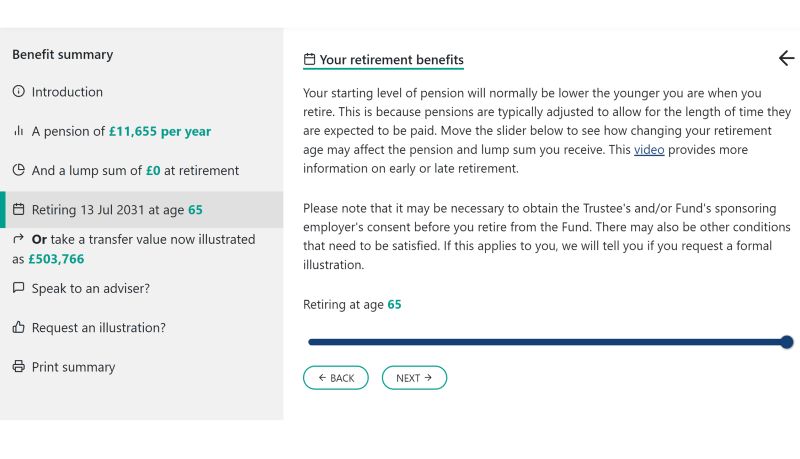### Detailed Caption:
In the provided image, the interface is divided into two main sections. On the left side, there is a sidebar under the heading "Benefit Summary" in bold text. The sidebar lists several options sequentially:

1. **Introduction**
2. **A pension of £11,655 per year**
3. **A lump sum of £0 at retirement**
4. **Retiring on 13 July (abbreviated JUL) 2031 at age 65**—this option is grayed out, indicating it has been selected.
5. **Or take a transfer value now illustrated as £503,766**

Below these options, there are additional actions: "**Speak to an advisor?**," "**Request an illustration?**," and "**Print summary**."

On the right side of the image, the main content area is titled "Your Retirement Benefits." Here, it explains that the starting level of pension will generally be lower the younger you are when you retire, due to adjustments for the length of time the pension is expected to be paid. Users are prompted to move a slider below this explanation to see how changing the retirement age affects the pension and lump sum they will receive. 

A hyperlink labeled "This video" (underlined in blue) offers more information on early or late retirement. 

The text further notes that it may be necessary to obtain the trustee's and/or the fund sponsoring employer's consent before retiring from the fund, with "Fund" capitalized. There could also be other conditions that need to be satisfied; if applicable, users would be informed upon requesting a formal illustration.

Towards the end, there is a mention of "Retiring at 65," with navigational options "**Back**" and "**Next**" buttons provided.